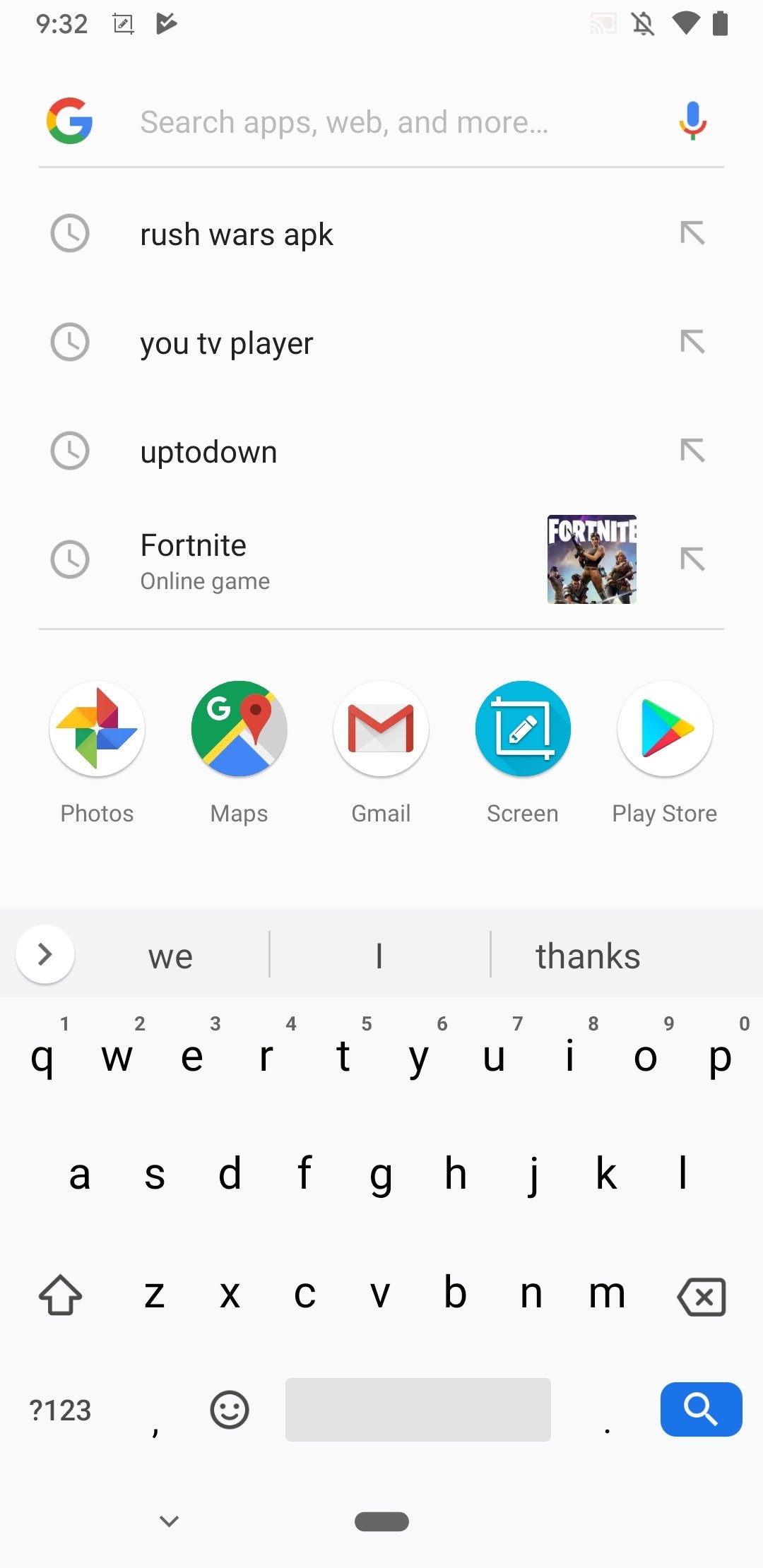This image is a detailed screenshot from a mobile device featuring a light gray, almost white, background for the entire screen. At the top of the screen, the mobile UI displays the time, "9:32," in dark gray on the top left. Next to the time, there is an unfamiliar icon resembling a square around an object, followed by another unfamiliar icon that looks like a triangle with a checkmark inside. To the right of these is a faintly visible icon, likely the cast icon, which appears very faded. The notification icon shows that notifications are disabled, followed by the Wi-Fi icon indicating an active connection, and the battery icon, arranged vertically and displaying a full charge.

Below this UI strip is the main content area that reflects the user’s current activity or screen. Here, a Google "G" logo is on the left, alongside a search bar that states "Search apps, web, and more..." with a voice search icon on the right, indicating this is a Google search interface on a mobile device.

Beneath this search bar is a section listing recent searches including “Rush Wars APK,” “UTV Player,” “Up 2 Down,” and “Fortnite.” Each search query is accompanied by a clock icon on the left and an arrow pointing northwest on the right.

Following the recent searches, there is a dividing line, and below it are various Google application icons, specifically Photos, Maps, Gmail, Screen (which is likely a screenshot tool, corresponding to the earlier unfamiliar icon), and the Play Store. Further down, the active layout of the Google keyboard, which was being used for typing, is visible at the bottom of the screen.